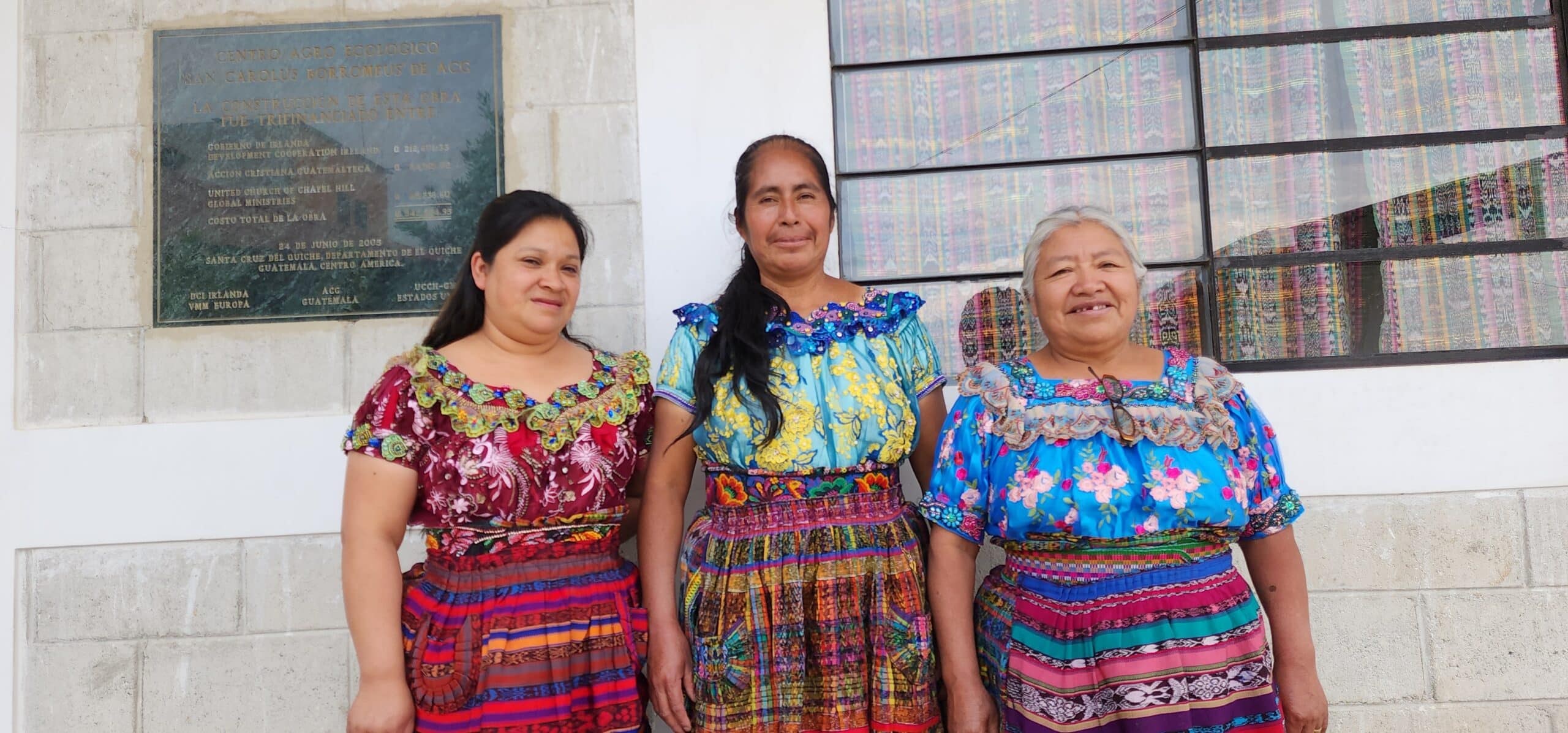Three Indigenous women, descending in age from left to right, stand outside a grayish-white stone building adorned with horizontal lines and an engraved green marble plaque reading "Centro Agios San Carlos, Castelotodo de la Ustra, Guatemala, Central America." The youngest woman on the left has long straight black hair pulled back slightly and is smiling. She wears a vibrant dark red floral top with green-edged ruffles and a colorful striped skirt. The woman in the center also smiles with long black hair, donning a light blue and yellow floral top with ruffles around the neckline and a bright patchwork skirt. The oldest woman on the right wears a turquoise shirt paired with a colorful striped skirt. They stand proudly in their bright and colorful attire, signifying their cultural heritage and familial bond as they pose against the predominantly stone gray backdrop of the building.